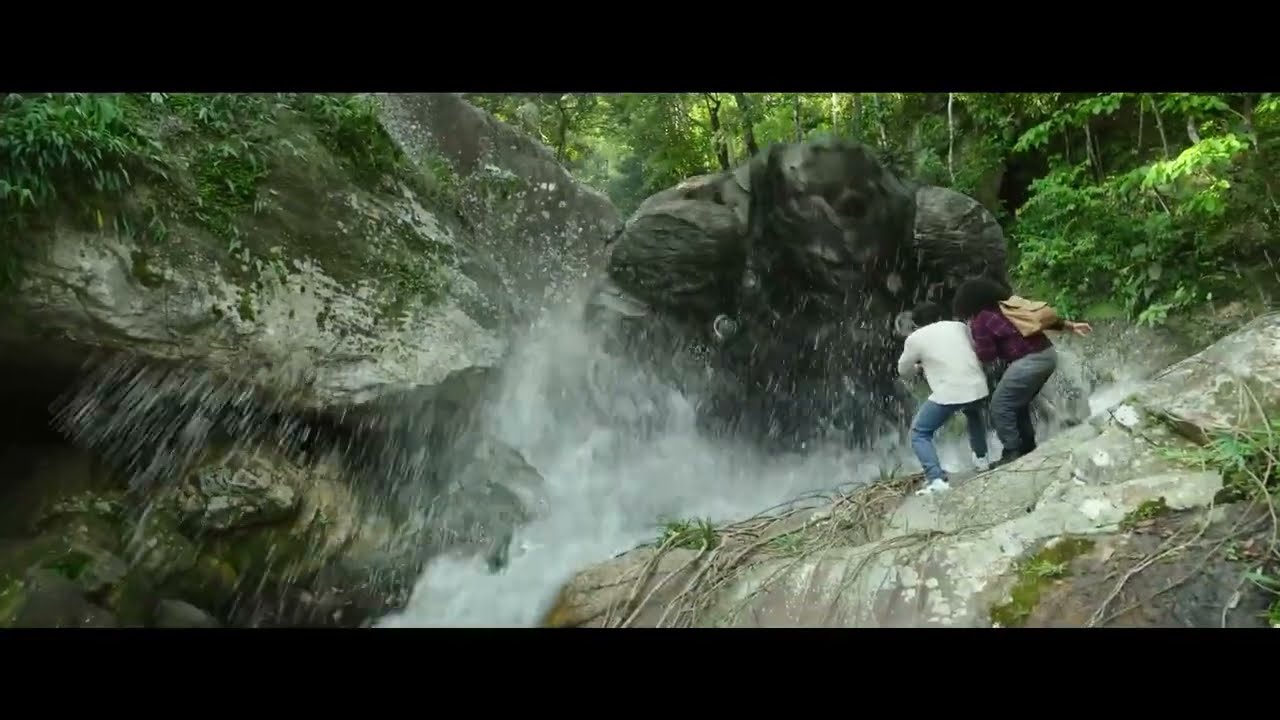In the picture, a man and a woman are crouched on a large boulder situated in the lower right corner of the frame, amidst a lush rainforest setting. The man, dressed in a white shirt, blue jeans, and white shoes, and the woman, in a purple shirt, grey slacks, and carrying a beige backpack, face away from the camera. Directly in front of them, rising from splashing water, is a gigantic, animated gorilla, its block-style CGI making it appear as though it has shoulders made of rocks. This figure is evidently fictional, likely from a film set, resembling an iconic movie scene such as King Kong. The scene is enveloped by a visible jungle backdrop, with more stone cliff formations and greenery on the left side, enhancing the dramatic encounter. The animation of the gorilla, coupled with the lifelike realism of the people and their surroundings, creates a striking contrast.